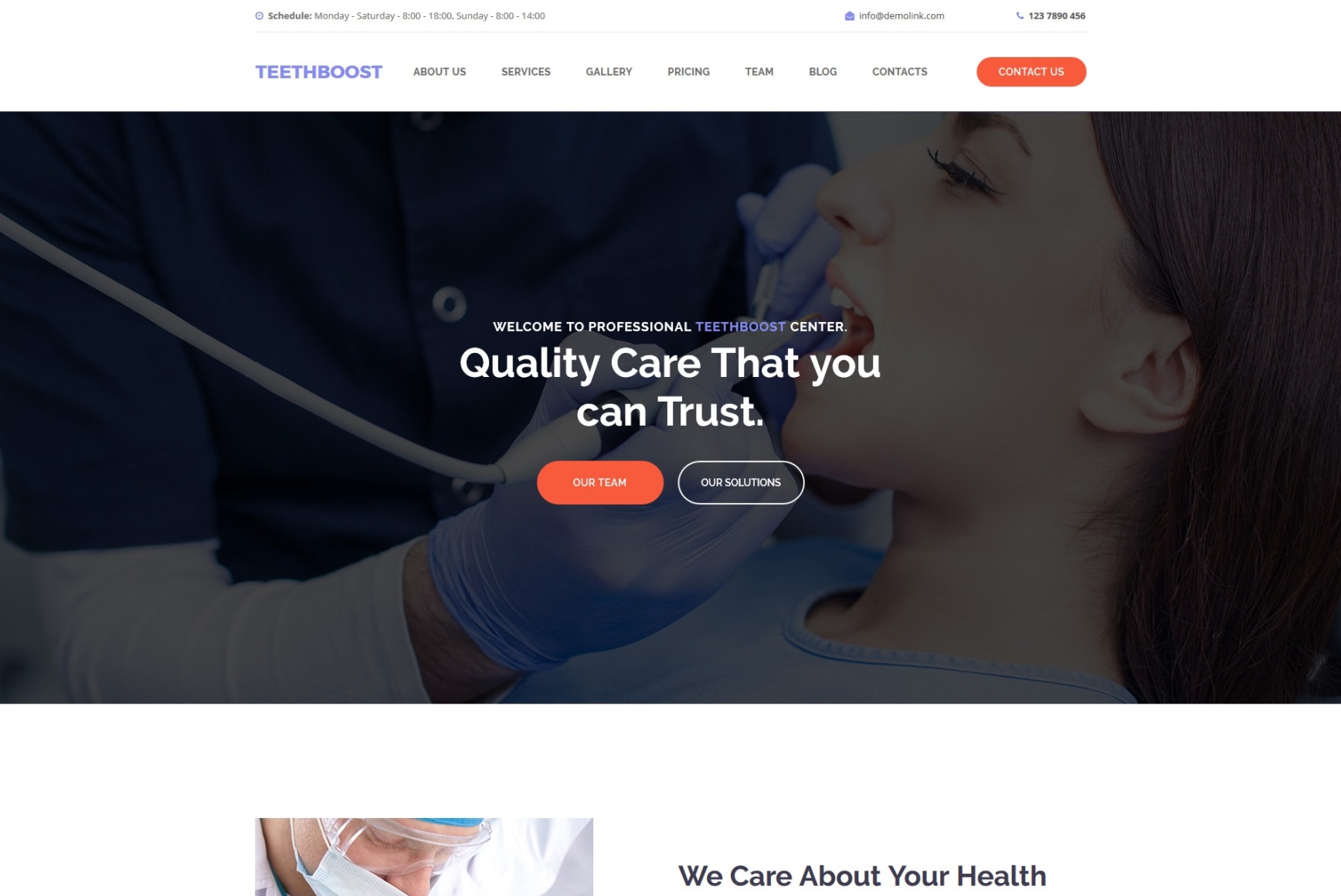A website screenshot showcasing the homepage of "Teeth Boost," a dental health company. At the top left of the header, which is white, is the company name, "Teeth Boost." To the right, the navigation menu includes tabs: About Us, Services, Gallery, Pricing, Team, Blog, and Contacts, along with an orange 'Contact Us' button. On the top right corner, there is a phone number preceded by an email address.

Below the header, the background image depicts a close-up of a dental patient undergoing an examination by a dental hygienist wearing purple gloves and holding a cleaning tool. Overlaid on this photo, the text "Welcome to Professional Teeth Boost Center" is prominently displayed, with "Teeth Boost" highlighted in purple and the rest of the text in white. Below this line, in larger white text, it reads, "Quality Care That You Can Trust." Positioned beneath this title are two call-to-action buttons: an orange 'Our Team' button on the left and an 'Our Solutions' button on the right.

Following a small gap below the main image, a smaller picture of a dental hygienist's face, masked and wearing goggles, appears. To the right of this picture, text in a matching theme reads, "We Care About Your Health."